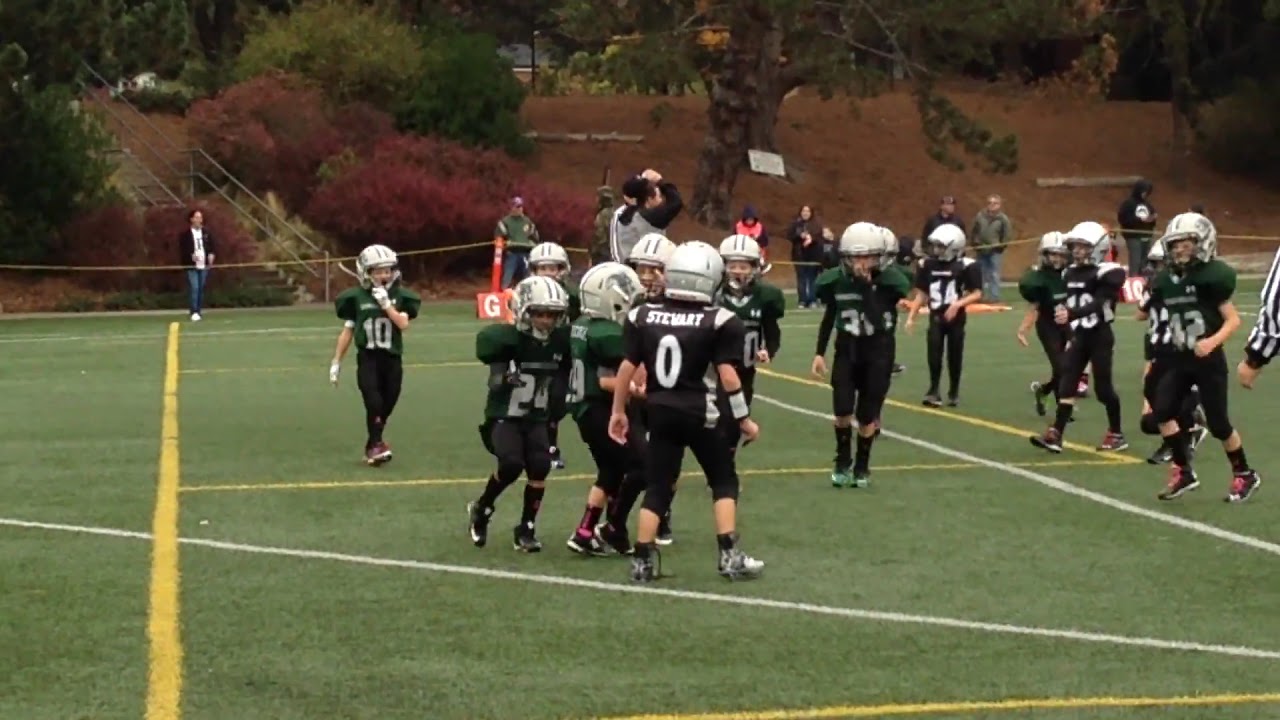In this vibrant outdoor photograph taken in the middle of the day, we see an energetic peewee football game in progress. The scene is set on a well-maintained AstroTurf field, marked with yellow and white lines. Centered in the image are young football players, their smaller statures suggesting they are children. Two teams are engaged in a scrimmage, with a referee positioned to the right.

The players are dressed in distinct uniforms—one team sports green jerseys with black pants, while the other team is in all black. Numbers are visible on the jerseys, such as 10, 24, 31, 42, and 54, with one player, Stewart, wearing number 0. The young athletes are equipped with cream-colored helmets, and their footwear includes combinations of black, red, white, and black and red socks.

Surrounding the field, there's a picturesque park area featuring lush greenery. At the top of the image, a staircase ascends a bank adorned with a mix of red and green bushes, leading up to a backdrop of trees with overhanging green foliage. A few man-made structures, including a pole and a possible building emitting a yellow glow behind the tree line, add to the backdrop complexity. This lively scene is encapsulated by spectators, bushes, and the clear blue sky, creating a spirited, communal atmosphere.